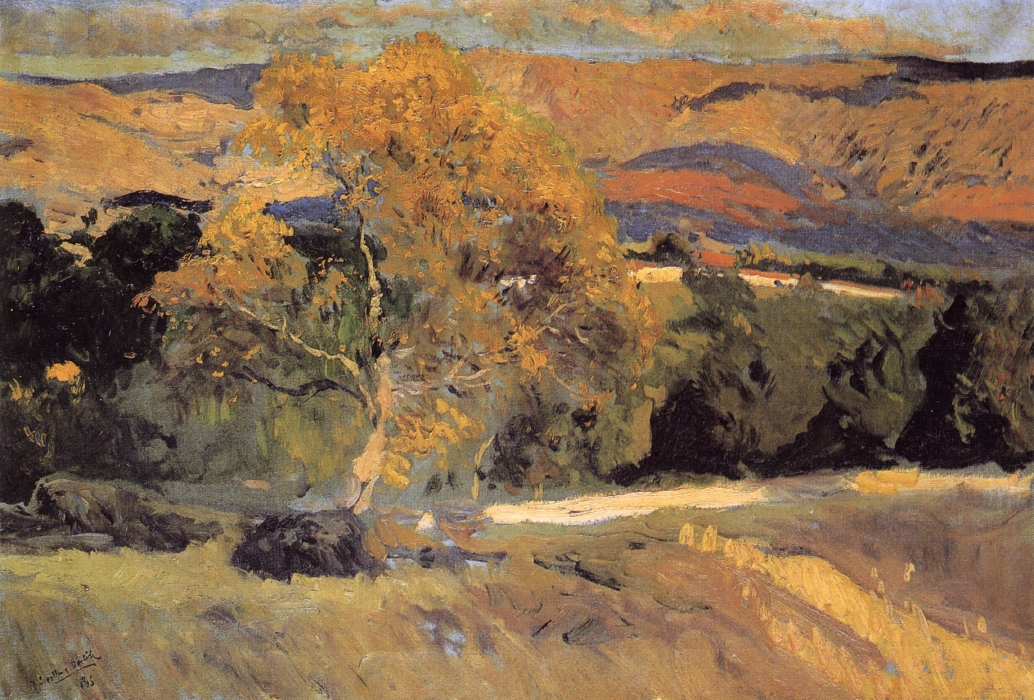This painting is an abstract depiction of a natural landscape, characterized by broad patches of color and explicit brush strokes. Dominating the scene is a large tree, positioned slightly to the left of the center, adorned with golden, yellow, and orange leaves suggestive of autumn. The tree stands on a terrain painted with a mix of yellow, brown, and green hues, indicative of grass and possibly a sandy path. Beside it are a couple of large rocks. Surrounding the main tree, especially in the middle and right-hand side, are shorter trees painted in dark to light green, adding depth to the landscape.

Behind these trees, the landscape transitions to rolling hills and mountains painted in a palette of brown, dark blue, purple, and red, creating a dramatic backdrop. Above the landscape, the daytime sky is a vivid blue filled with clouds tinged in orange, yellow, and light green, which may suggest a late afternoon or early evening ambiance. The lower left corner of the painting bears the signature of the artist, adding a personal touch to this vivid, textured scene.